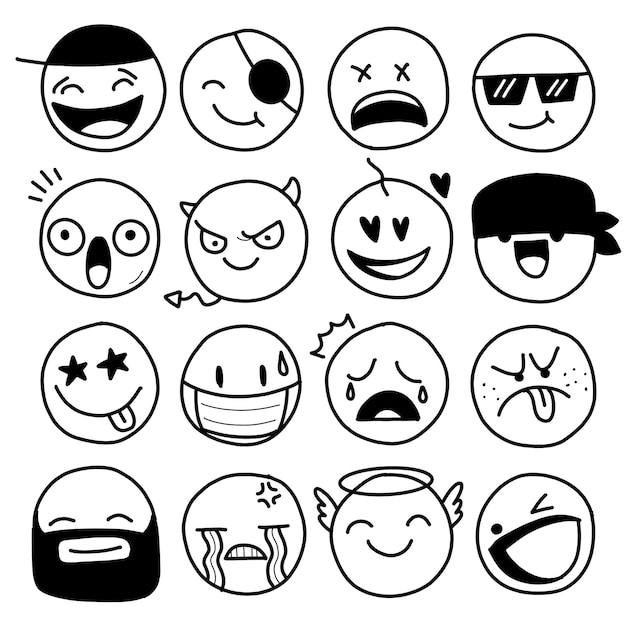The image is a black and white line art illustration showcasing 16 emoji-like faces arranged in a 4x4 grid format. Each face is a simple circle with no additional features like hair or ears but has varying expressions and accessories drawn inside. The faces exhibit a range of emotions, some happy, some sad, and others in between. Notable details include a top left emoji that is smiling with its eyes closed, mouth open, and a black cap tilted sideways; another emoji with a closed eye and a black eye patch next to it; a frowning emoji with its mouth open and two X's for eyes; and one wearing black sunglass shades. Further down, there is an emoji with angel wings and a halo, another with a tongue sticking out, one crying, and one masked. Some emojis have simple dot eyes while others have more detailed eyes with pupils. The image captures a playful, cartoon-like quality reminiscent of stick figure art, emphasizing humor and a variety of emotional expressions.